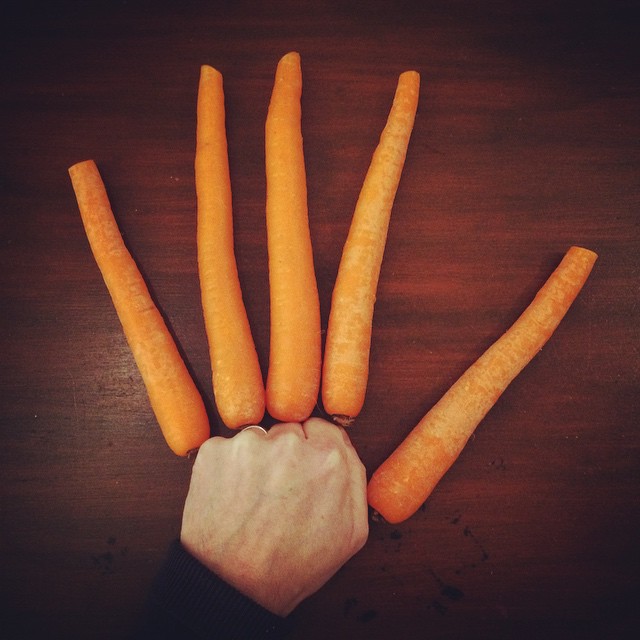The image features a detailed, artistically rendered photograph set against a dark red, woodgrain countertop. At the center, a man's left fist extends from the bottom middle of the frame, slightly to the left. His skin is white, and he wears a wedding band on his ring finger. The fist is tightly closed, with the fingers folded underneath, replaced by five carrots extending outward from each knuckle. The bright orange carrots have a rough texture and flat ends, mimicking the appearance of fingers, with the thumb carrot unusually long, nearly matching the length of the other four. The overall tone of the square image is warm yet low in saturation, highlighting the intricate details of both the fist and the mahogany or cherry wood-patterned table beneath it. The composition and unique vegetable embellishment evoke an imagery reminiscent of Wolverine's iconic claws, possibly suggesting themes of strength or an artistic take on everyday objects.